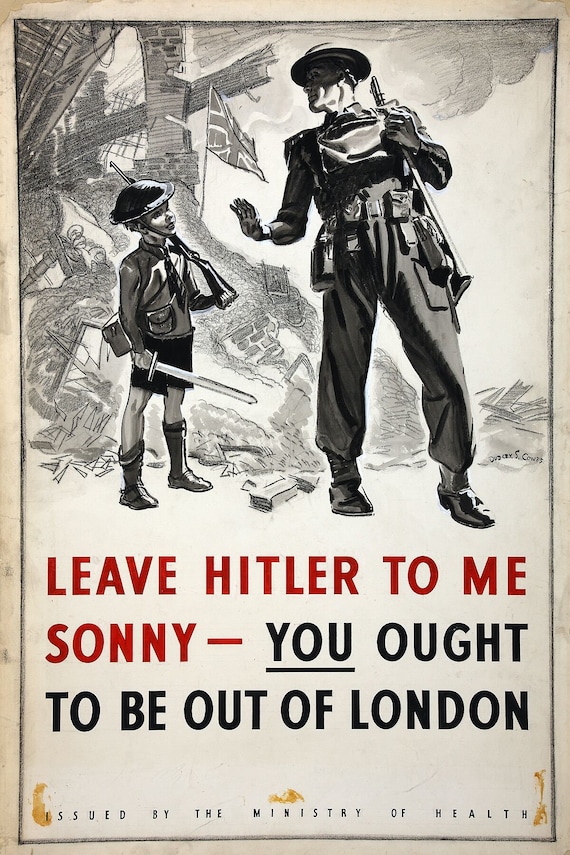This World War II poster, issued by the Ministry of Health, features a striking visual composition rendered in black and white with accents of red. Dominating the center is a British soldier in full uniform, carrying a rifle, and seemingly engaged in a poignant dialogue with a young boy. The boy, dressed in knee socks and bearing toy weapons—both a rifle and a sword—appears ready for combat himself. Above them, the bold red text commands, "Leave Hitler to me, Sonny," while in smaller black letters, the urgent directive follows, "You ought to be out of London," with "You" emphatically underlined. The text, all in capital letters, drives the wartime message home.

Behind the pair, one can see the bleak consequences of the conflict: buildings reduced to rubble, likely from German bombings, with plumes of smoke still lingering. Amidst the destruction stands the resilient symbol of the British Union Jack flag, protruding defiantly from the debris. This powerful scene encapsulates the wartime spirit, with a protective soldier urging the evacuation of children from the ravaged city—taking up the fight himself so the young can seek safety.